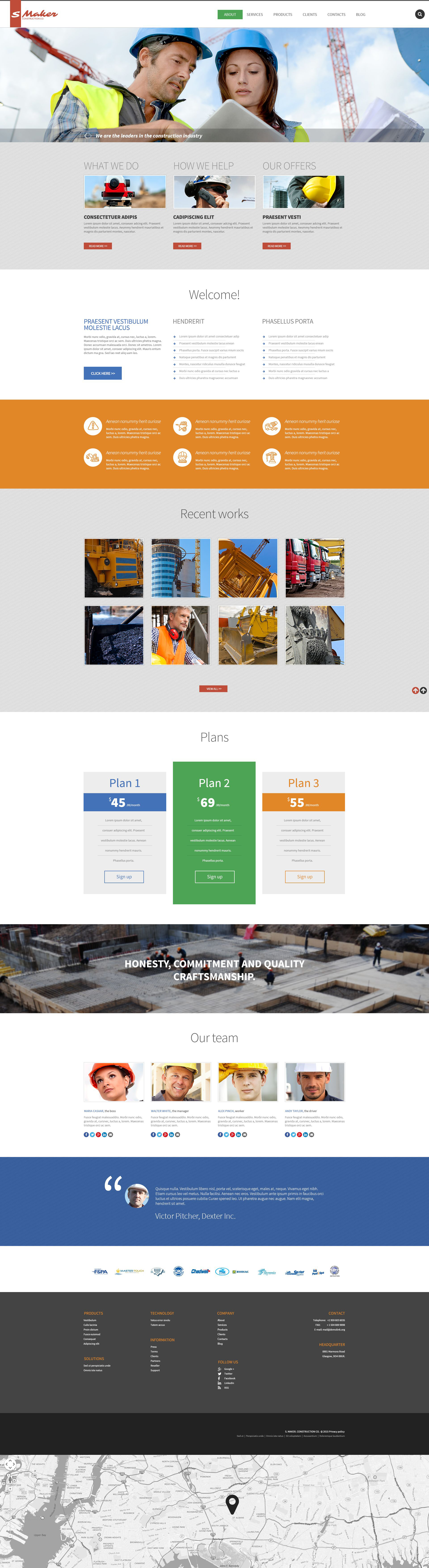This screenshot captures the homepage of the website for a construction company called S Maker. The image appears to be somewhat blurry and stretched, necessitating significant zooming to clearly view the content. The homepage layout is versatile and encapsulates the entire screen.

In the top left corner, the company's logo, "S Maker," is prominently displayed, indicating it specializes in the construction industry. On the top right, there is a navigation menu featuring buttons labeled "About," "Services," "Products," "Clients," "Contacts," and "Blog," accompanied by a magnifying glass icon for the search function.

Beneath the navigation menu spans a large horizontal image of a male and female construction worker examining what appears to be a blueprint or plan. This imagery is accompanied by the slogan, "We are the leaders in the construction industry." 

Further down the page, the content is divided into several sections with headers in English such as "What We Do," "How We Help," and "Our Offers.” Additionally, there is a "Welcome" section, though the accompanying descriptive text is in an unfamiliar language. Another notable section titled "Recent Works" displays various images illustrating the projects the company has completed. 

This comprehensive homepage succinctly communicates the company's expertise and services while providing visual evidence of their recent accomplishments.